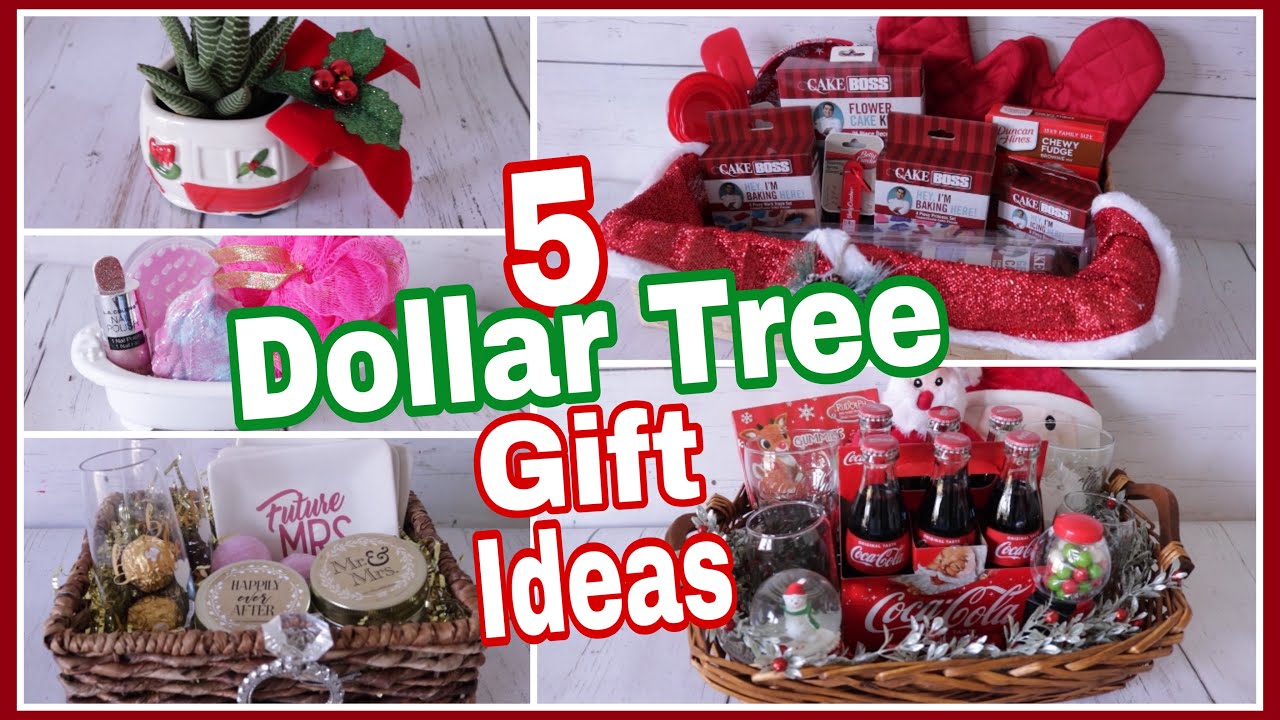The image showcases a vibrant advertisement titled "Five Dollar Tree Gift Ideas," with the words "Dollar Tree" surrounded by a green outline. The number "5" is in white, outlined with a red border, and "Gift Ideas" is also in white with a red border. There are five distinct gift ideas presented as photos arranged in a pattern — three on the left and two on the right.

1. **Top Left:** A festive flowerpot featuring a poinsettia adorned with a red ribbon and green leaves with red berries.
2. **Middle Left:** A succulent in a ceramic bowl with a red ribbon, nestled among some bath essentials including a scrubby and a foot brush.
3. **Bottom Left:** A basket labeled "Mr. and Mrs." with various candles, including a "Future Mrs." candle and a hurricane candle holder.
4. **Top Right:** A red and white basket filled with Cake Boss products and oven mitts.
5. **Bottom Right:** A collection of Coca-Cola-themed gifts, featuring glass Coke bottles, a Coca-Cola snow globe, and a Santa toy.

These gift ideas are perfect examples of budget-friendly yet thoughtful presents available at Dollar Tree, ideal for holiday giving.